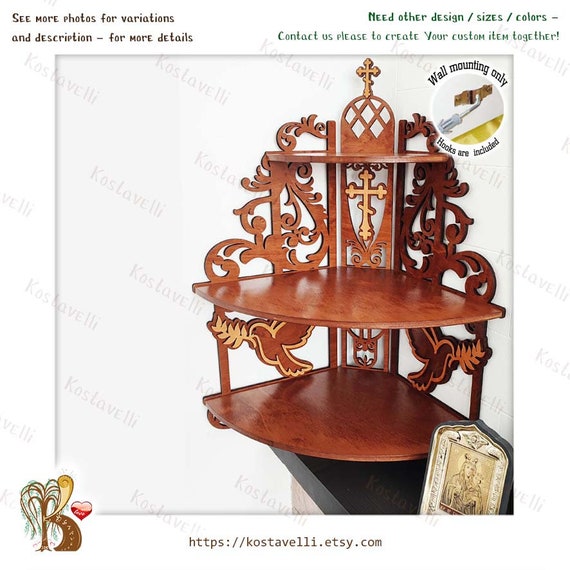This is an advertisement image for an ornate, religious-themed wall-mounted shelf, likely being sold on an Etsy shop. The shelf, crafted from dark or red wood, features three intricately carved levels that can hold ornaments, candles, or other decorative items. Each tier is adorned with religious symbols, including crosses, doves holding olive branches, and floral designs, giving it a distinguished and devout appearance. 

The photo includes a watermark with "Costa Valley" written diagonally across the white background, and a small tree illustration in the bottom left corner. There is also a gold logo on the bottom right. Text boxes are located at the image's bottom left and right, providing details on options for customization and a website link to purchase the item. Additional information above the image instructs viewers to see more photos for variations and further descriptions. This elegant piece serves both as a functional shelf and a religious display, perfect for those who appreciate artful craftsmanship and spiritual decor.